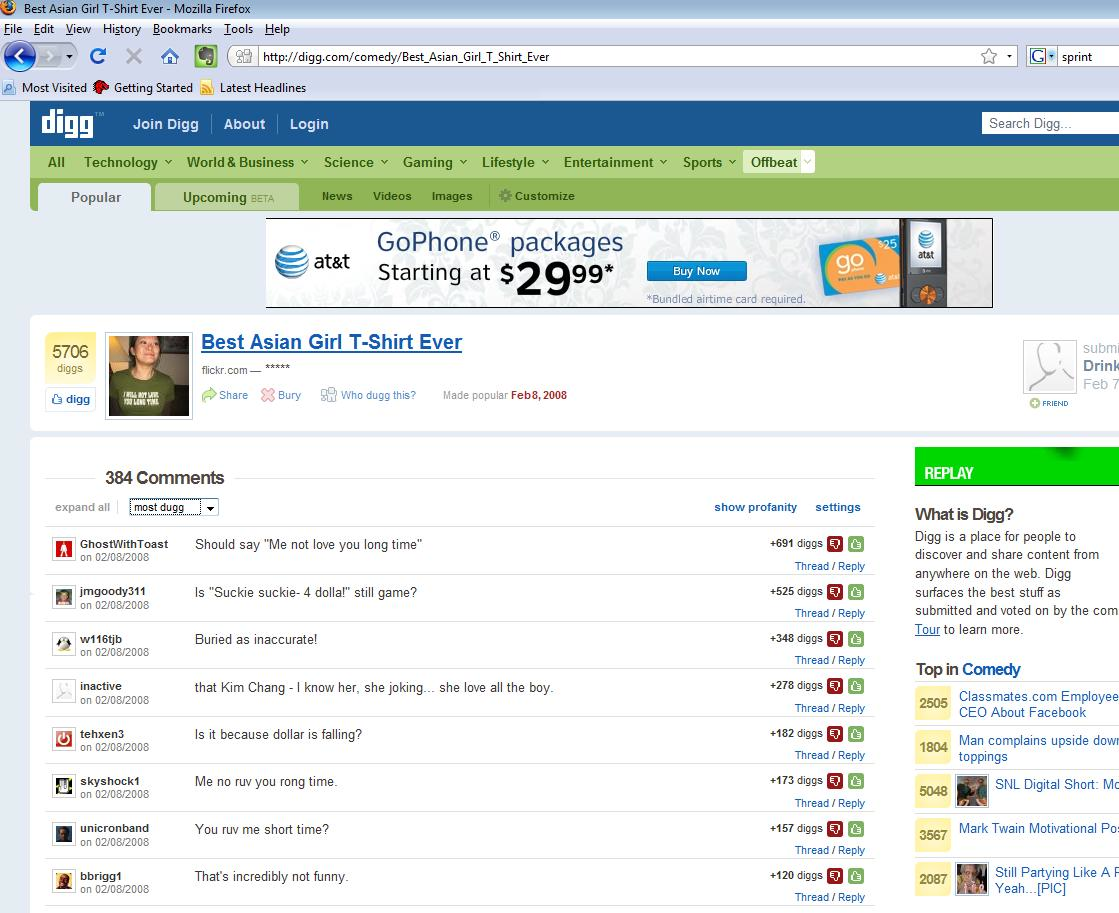In this screenshot, we see a webpage open in a Mozilla browser. The browser interface shows standard menus (File, Edit, View, History, Bookmarks, Tools, Help) at the top. The URL in the address bar reads "http://dig.com/comedy/best_asian_girl_t-shirt_ever."

The webpage is from the website Dig, evident from the "Dig" logo in the upper left corner. Next to the logo are navigation links for "Join Dig," "About," and "Login." Below these links is a green header with dark green text containing various categories: All, Technology, World & Business, Science, Gaming, Lifestyle, Entertainment, Sports, and Offbeat.

The main content area is open to the "Popular" section, showcasing an item titled "Best Asian Girl T-Shirt Ever." The focus of this section is an image of a girl wearing a green t-shirt. To the right of the image is a credit to "flickr.com." Below the t-shirt image, there is a count indicating 384 comments have been made about this post.